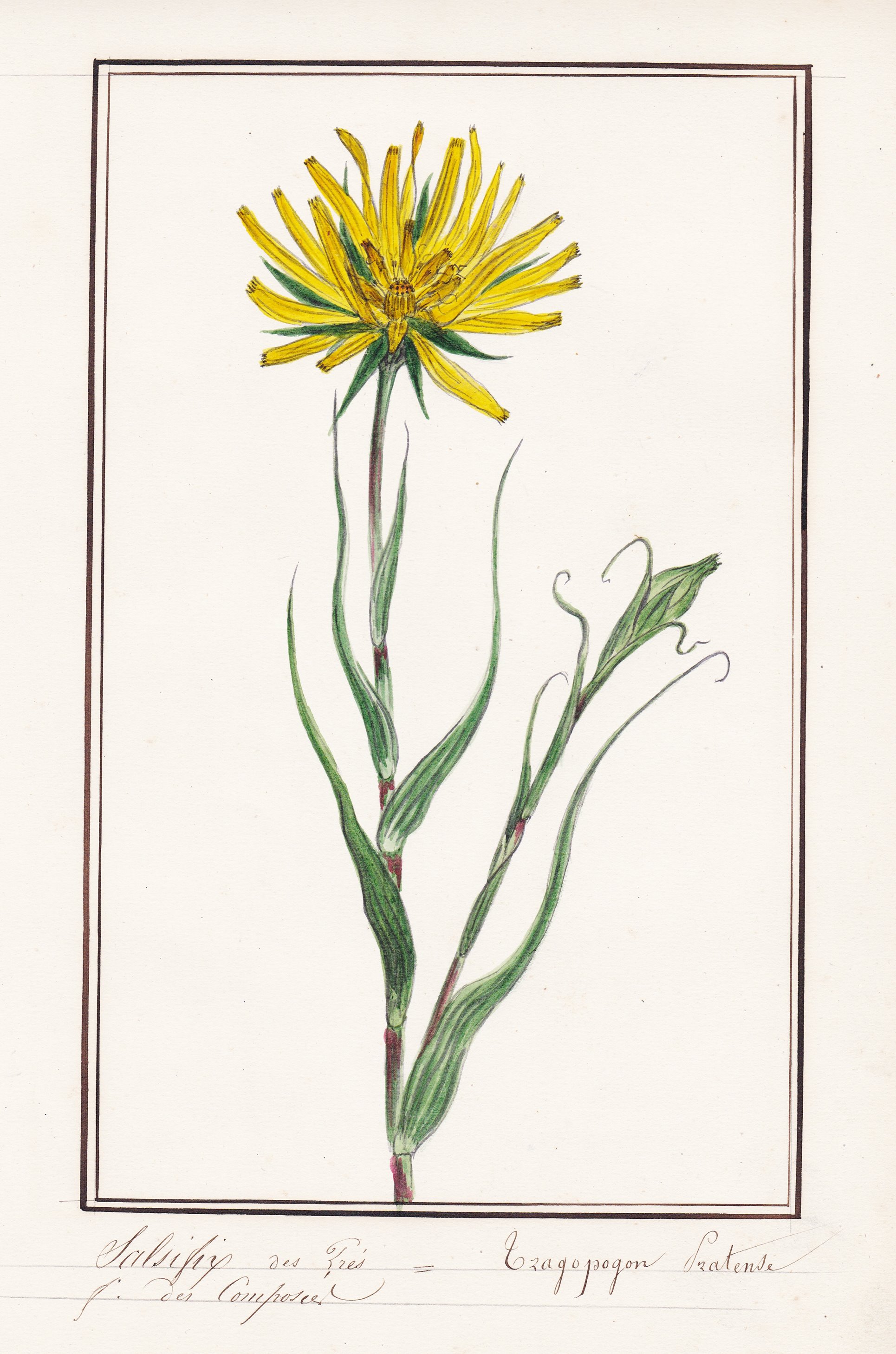This image is a rectangular, vintage-style poster with dimensions taller than it is wide. The poster is ivory-colored with a brown, hand-drawn rectangle framing a detailed illustration of a tall, yellow flower. The flower has long, thin, wispy petals in a burnt yellow hue. Its stem is brown, adorned with many slender, green leaves, some tinged with red. These leaves extend both upward and downward along the stem. Surrounding the flower is a thin black border, followed by an even thinner inner black border. Below the illustration, in cursive scripting that appears difficult to decipher and possibly in another language, is a two-line engraving. The minimalist background draws focus to the intricate flower and the delicate cursive writing beneath it, making the entire composition visually striking.